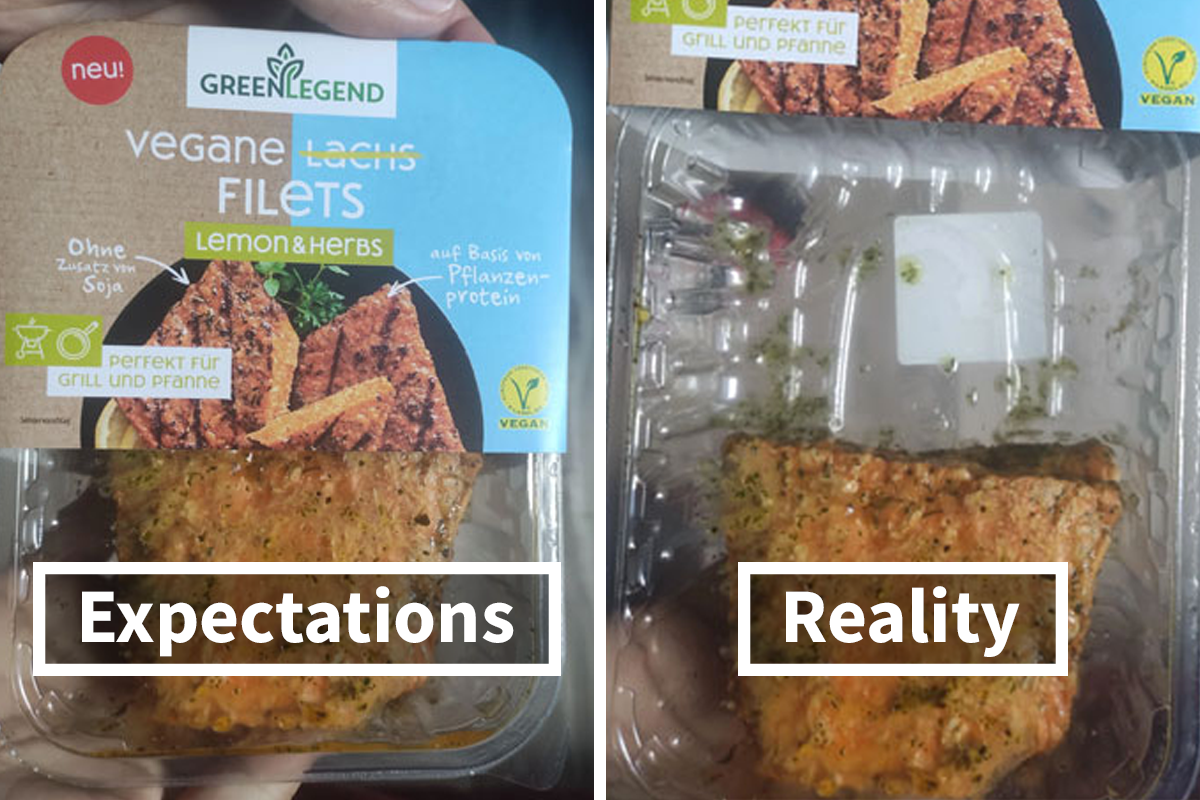The image is a humorous side-by-side comparison showcasing the discrepancy between the advertised and actual product contents. On the left side, labeled "Expectations" in large white letters, there is the packaging of Green Legend Vegan Fillets with Lemon and Herbs. The packaging, partially transparent, reveals what looks like two hearty, seasoned fillets ready for grilling or frying. The cardboard label features bright visuals and text predominantly in German—"NEU" (New) in a red circle and mentions of it being vegan. This creates the impression of a full and appetizing product.

On the right side, labeled "Reality" in the same font, the image shows the packaging with the cardboard cover lifted. This reveals that the actual contents fall far short of the expectation, with only half of the plastic container being filled—lacking the enticing garnishes and appearing less appealing. The container tricks the viewer into expecting it to be fully packed, but in reality, it is disappointingly half-empty. This contrast starkly highlights the difference between marketing visuals and the true product, capturing the essence of expectation versus reality in a visually engaging and relatable manner.